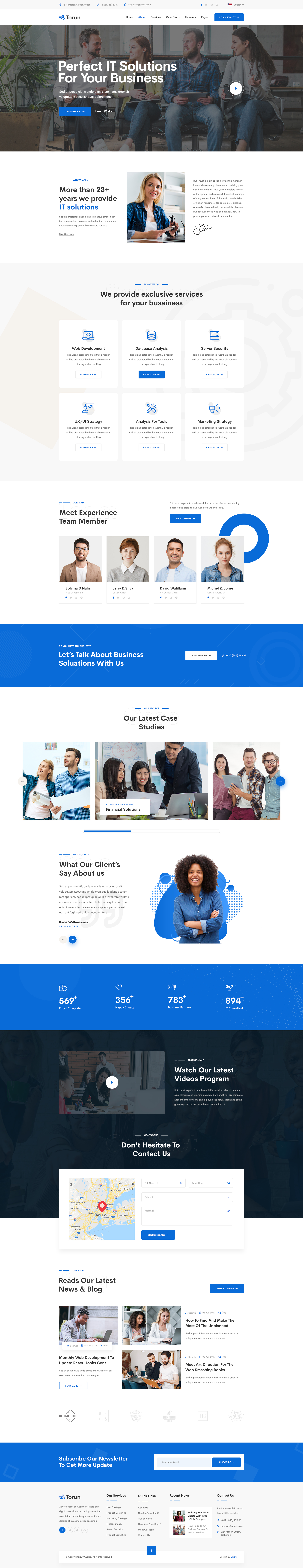The image is a detailed collage of multiple website screenshots, arranged in a manner that mimics a scrollable homepage. The layout includes around five to seven pages compressed into a single image, making the text hard to read. However, the visible content indicates that the website is for an IT solutions provider, as evidenced by the motto: "Perfect IT solutions for your business." The collage features numerous stock images depicting diverse groups of people working collaboratively in office environments, all appearing content. In addition to these images, there are several infographics and statistical data sections. The overall design of the website utilizes a clean, organized aesthetic with a predominantly blue and white color scheme.